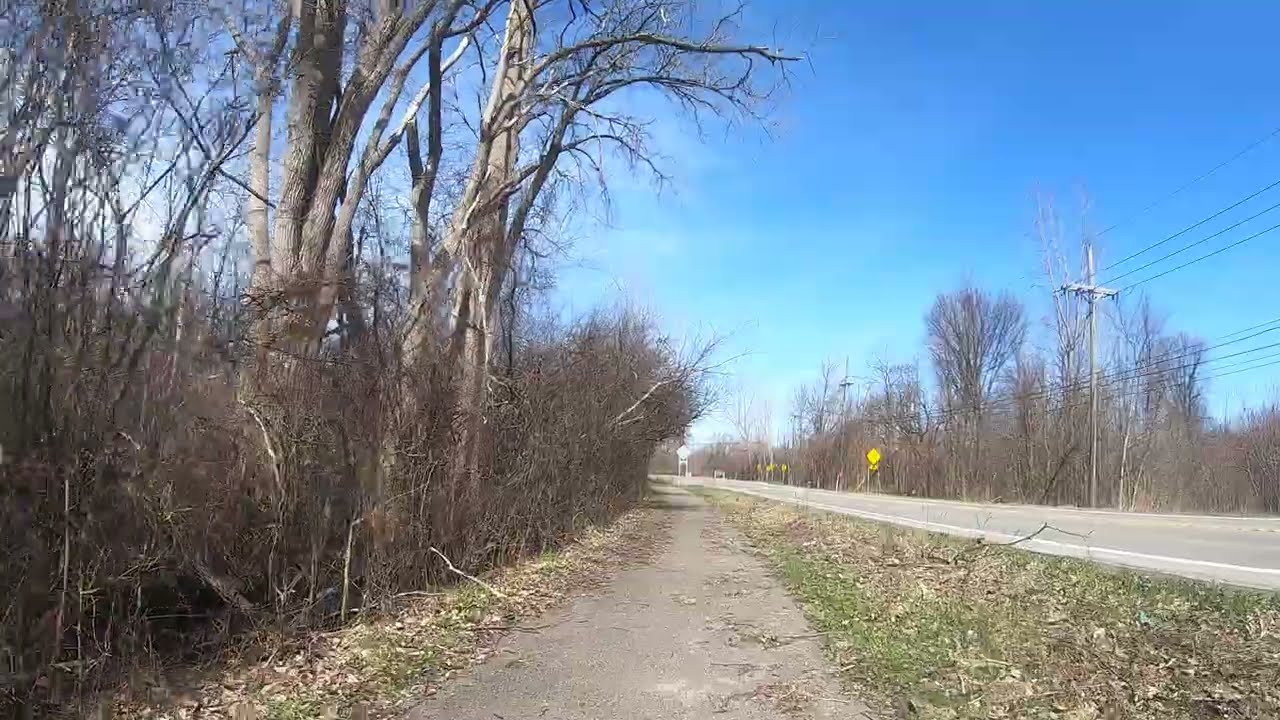The image depicts a tranquil outdoor scene featuring a concrete walking path that runs parallel to a two-lane highway. The highway, running to the right of the concrete path, is bordered by a strip of grass littered with fallen leaves, giving the impression of late autumn or early winter. The path itself, though rough-edged, seems well-worn and serene. To the left of the path, a dense array of leafless bushes and trees stand, their bare branches weaving a stark natural tapestry against the sky. 

On the right side of the highway, a series of telephone poles with intricate webs of electrical lines extends into the distance. Three yellow signs punctuate the roadside, hinting at some form of caution or instruction for oncoming drivers. The highway itself is marked with white stripes on the edges and a central yellow dividing line, clearly delineating the two lanes.

As the road stretches forward, it gently curves and eventually veers sharply to the left, disappearing from view. Overhead, the sky is a crisp blue, adorned with scattered white clouds primarily gathered to the right side of the photo. The absence of traffic and the quiet surroundings suggest a countryside setting, adding to the overall feeling of tranquility.